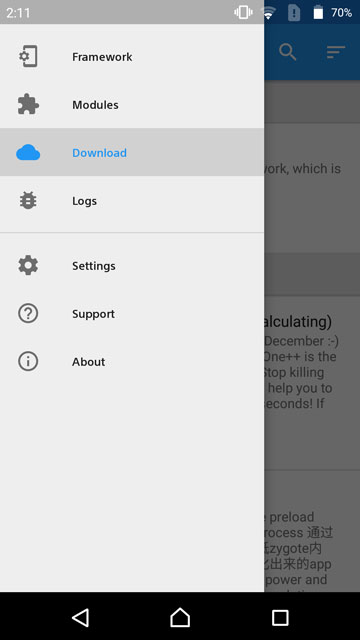The image is a screenshot of a mobile phone displaying a view of an application or website interface. The background color of the interface is gray, adorned with a darker gray banner at the top. In this banner, the time is shown as 2:11, and it indicates a weak Wi-Fi signal along with a battery level of 70%.

The layout includes several icons and options arranged in a row. The first icon is a rectangle labeled "Framework," followed by a puzzle piece icon named "Modules." Next is a blue cloud icon labeled "Download," which is highlighted in blue, signifying it is the currently selected option. Then, there is a bug icon titled "Logs," a gear icon named "Settings," a question mark icon for "Support," and an exclamation mark icon along with a circle labeled "About."

At the bottom of the screen, there is a black banner containing navigation icons: a back arrow, a home icon, and a square icon. This structured interface appears to belong to an application designed for managing various functionalities and settings.